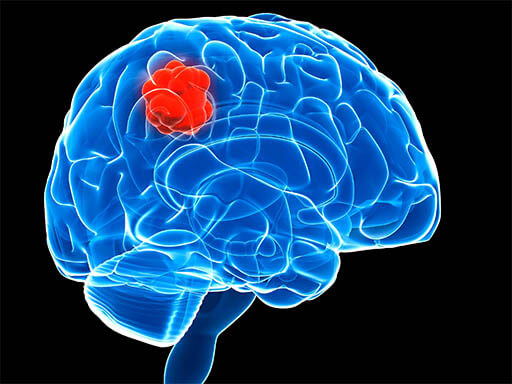The image depicts a computer-generated 3D model of a human brain on a solid black, square-shaped background. The brain is rendered in a vibrant blue color with intricate white outlines that illuminate the brain's detailed pattern of ridges and folds. Notably, there is a small cluster of glowing red cells located on the upper left side of the brain, which stands out starkly against the blue and white coloration, potentially indicating an abnormality, such as a tumor. Extending downward from the center at the bottom of the brain is a thin, darker blue handle, which seems to connect to the brain stem area. Adding an irregularity to the design, there's an irregular shape protruding from the bottom left part of the brain, enhancing the diagrammatic intricacy of the illustration.